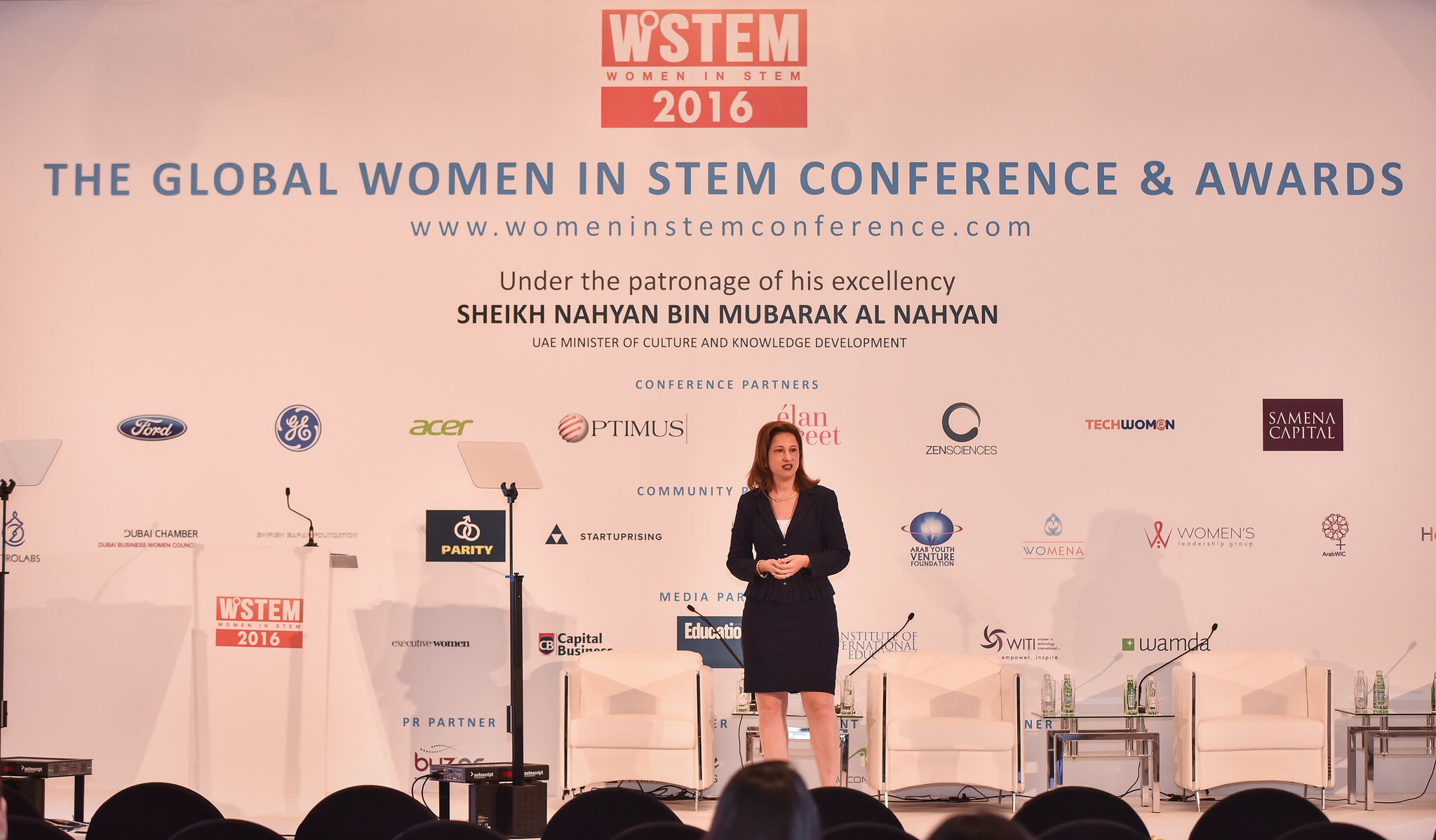The photograph depicts a woman giving a presentation on a stage, taken from the audience's perspective. She stands in the center of the image, a Caucasian woman with medium brown hair, dressed in a black skirt and suit jacket with a white shirt underneath. She has stepped away from the microphone and is addressing the audience with her hands folded in front of her. Behind her, the entire back wall of the stage is a solid white backdrop featuring multiple lines of text and logos. At the top center is a red rectangular logo that reads "WSTEM" in white font, with a white banner running through it that says "Women in STEM," and the numbers "2016" beneath it. The blue text across the center states, "The Global Women in STEM Conference and Awards, www.womeninstemconference.com." Below, in black text, it reads, "Under the Patronage of His Excellency Sheikh Nahyan bin Mubarak Al Nahyan, UAE Minister of Culture and Knowledge Development." The bottom of the photo shows the heads of audience members, while three empty chairs are visible on the stage. The setting appears to be an indoor conference event.